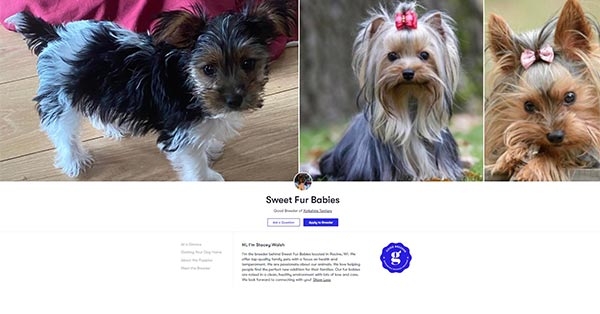Caption: "A welcoming header image of a group page titled 'Sweet Fur Babies' showcases three adorable dogs. On the upper left, a small dog with a unique black, white, and brown coat stands on a light oak-colored hardwood floor. A maroon blanket subtly adds to the cozy setting in the background. Next to it, a fluffy dog with long blonde fur and a pink bow sits gracefully in front of a tree, contrasting its darker gray body fur. To the right, another dog with reddish-brown fur and a pink bow lies comfortably on its front legs, creating a full-frame portrait. Below the images, the group name 'Sweet Fur Babies' is prominently displayed, accompanied by a stamp-style logo in blue featuring a white 'G'. Further textual details, though visible, are too small to decipher."